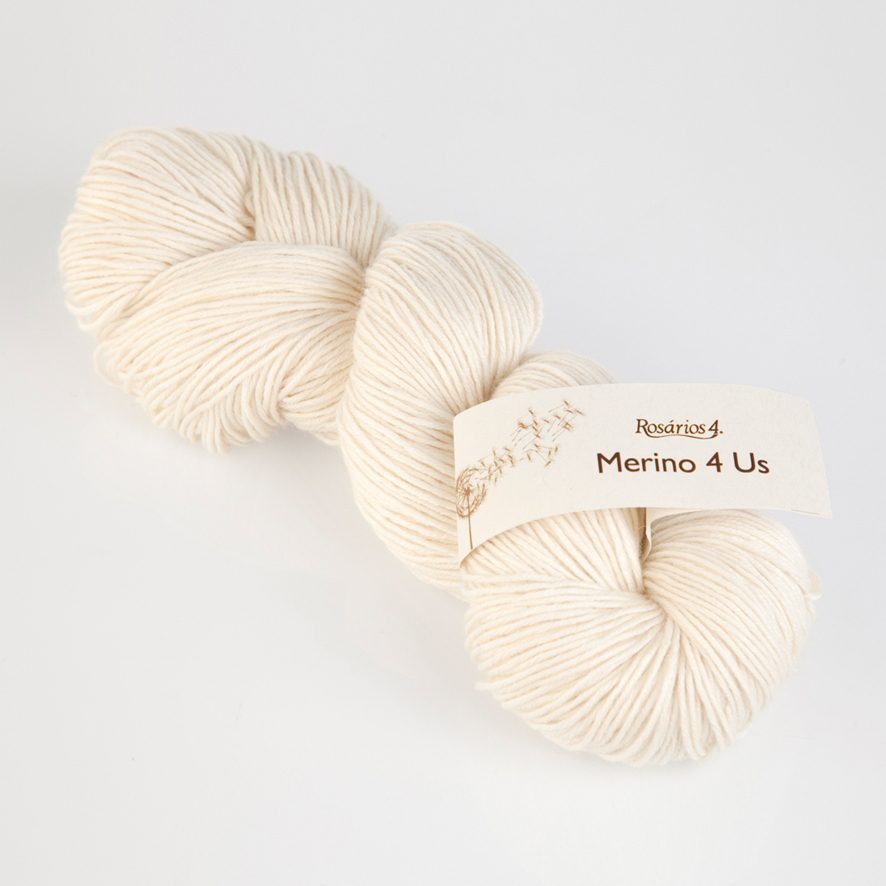The photograph showcases a skein of off-white, light brown merino wool, neatly looped into a figure-eight shape on a pale blue surface, likely indoors. The wool is adorned with a small, white tag featuring a stylized logo of birds or dandelion seeds blowing in the wind, illustrating a sense of delicate motion. The tag reads "Rosario's 4 Merino for us" in a darker almond color, providing a rich contrast against the light background. This carefully arranged skein, possibly for sale, reflects a meticulous and appealing presentation of high-quality merino wool.